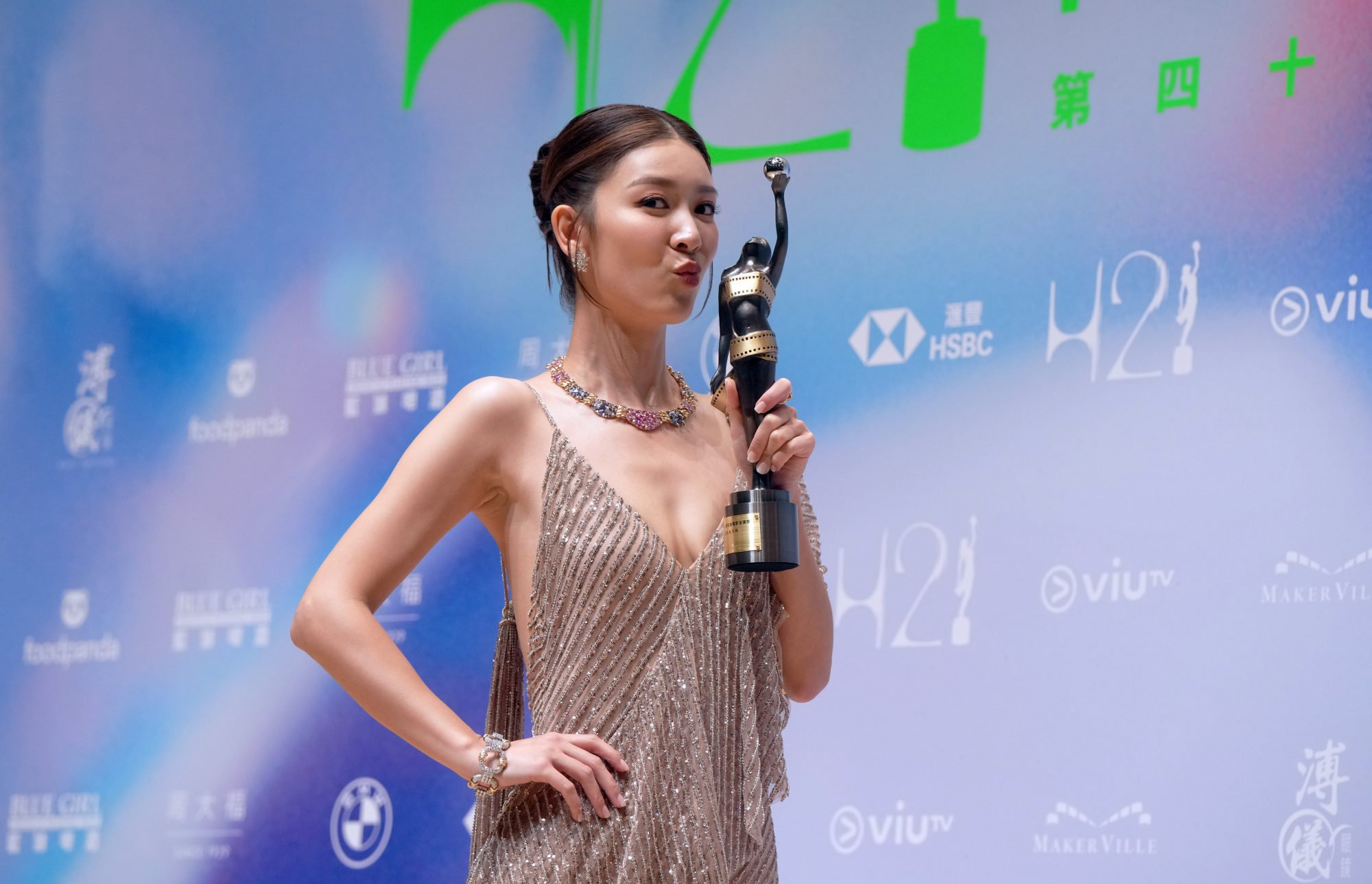The photo features an Asian woman, possibly a renowned actress or athlete, posing at an award ceremony on a step-and-repeat backdrop. She is clad in a silvery-beige evening gown with a deep V-neck and deep arm slits, accessorized with a striking statement necklace and a chunky gold bracelet on her right wrist. Her black hair with brown streaks is styled in an elegant updo with strands cascading down the sides of her face. She is holding a black and gold trophy featuring an outfit made to resemble camera film, and she is playfully making a kissy face towards it. The backdrop behind her features various brand names and sponsors in white text against a backdrop of blue, green, and rainbow holographic hues. The overall impression is one of glamour and celebration, highlighting her potential achievement in the field of entertainment or sports.